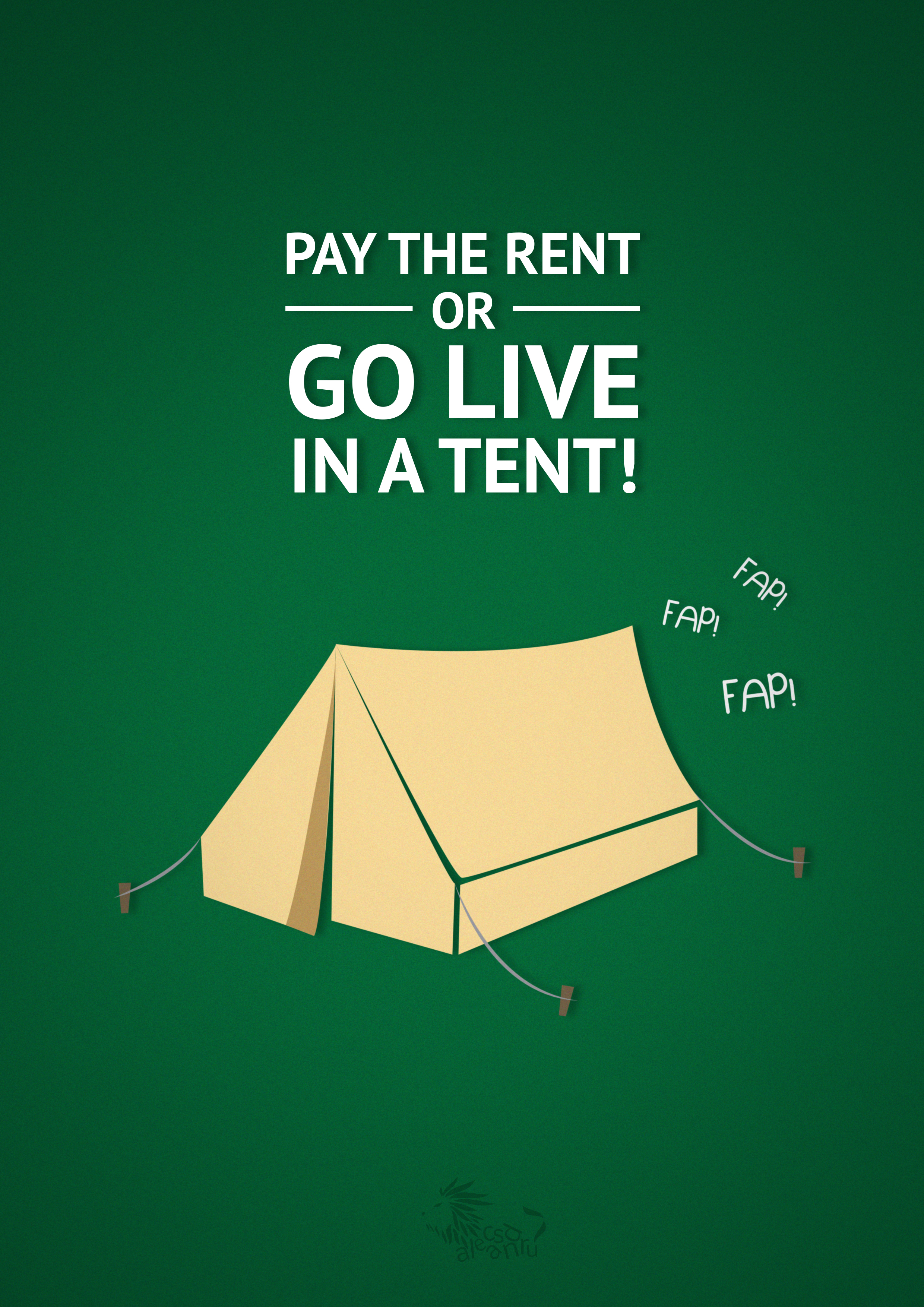This computer-animated image, which has the appearance of a poster or meme, features a green rectangular background with prominent white text at the top that reads "PAY THE RENT OR GO LIVE IN A TENT!" In the center below the text, there is a detailed illustration of a light yellow or tan-colored camping tent, complete with poles and connecting lines securing it to the ground. To the right of the tent, the word "FAP!" is repeated three times in white letters with exclamation points. The sign exudes a snarky and potentially insensitive humor, targeting the issue of homelessness.